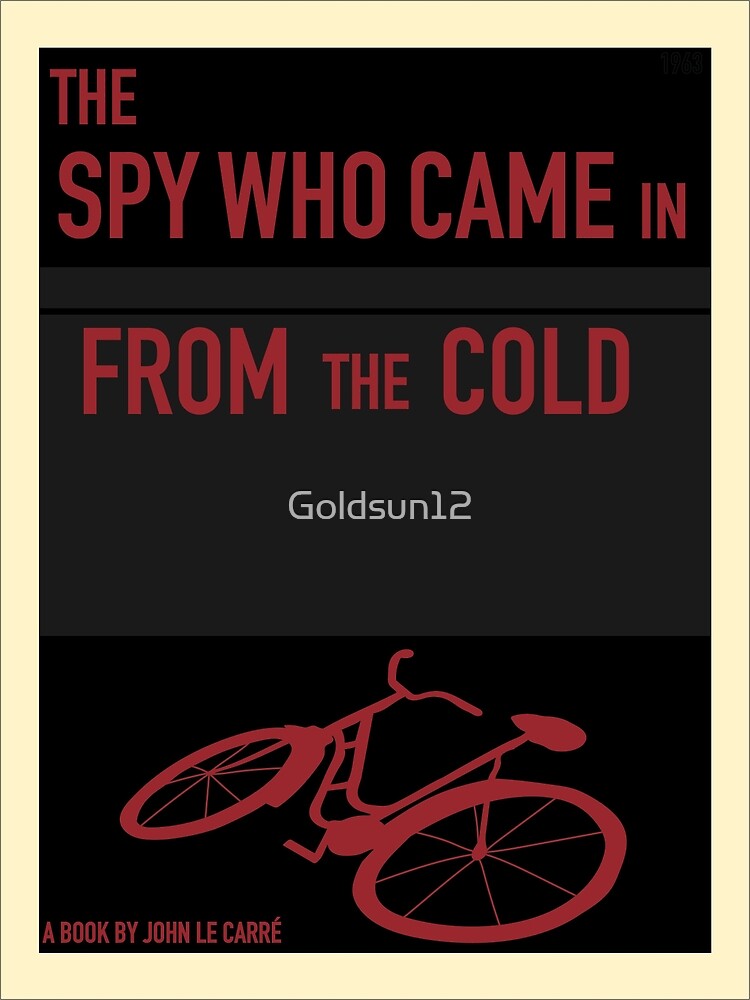The book cover for "The Spy Who Came In From The Cold" by John Le Carre features a striking design with a predominantly black background. The title is prominently displayed at the top in large red text, with the smaller words "the" and "in" interspersed among the larger text but still in red. Centrally placed in the middle section, which is a dark charcoal gray separated by a thin black line at the top, is a white text reading "Gold Sun 12." At the bottom left, there is a smaller red text declaring "A BOOK BY JOHN LE CARRE." A stylized, red silhouette of a bicycle lies on its side in the lower section of the cover. The entire design is bordered by what appears to be an ivory or yellowish frame, adding a subtle contrast to the overall dark theme of the cover.